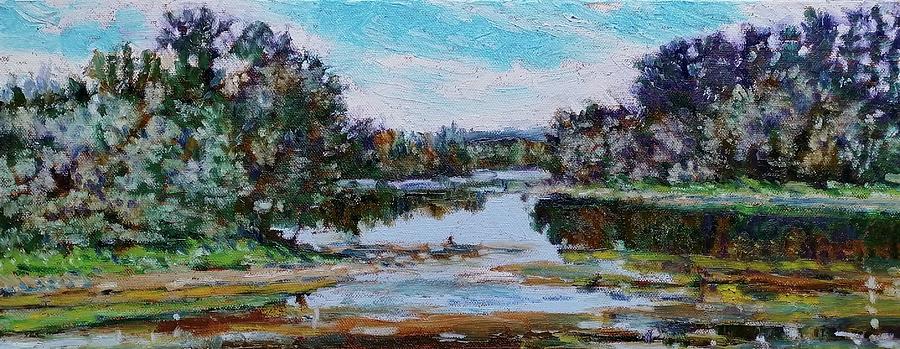This image showcases a large, rectangular watercolor painting in a landscape orientation, portraying a serene, abstract outdoor scene. Dominating the center is a body of water, potentially a pond or lake, curving to the right and ringed by greenery. The water's blue hues are interspersed with reflections of surrounding green, black, and tan trees, as well as yellow and brown streaks. The shorelines are varied: in the foreground, a marshy area leads into brown dirt at the bottom left, transitioning to a grassy knoll with trees to the right. Both the left and right banks are dense with foliage, dotted with dark and light splotches in an impressionistic style akin to Monet or Manet. In the distance, the horizon features a bright blue sky with wispy white clouds. The entire scene is rendered in broad, blotchy strokes, adding a hyper-unrealistic, abstract quality to the overall view.